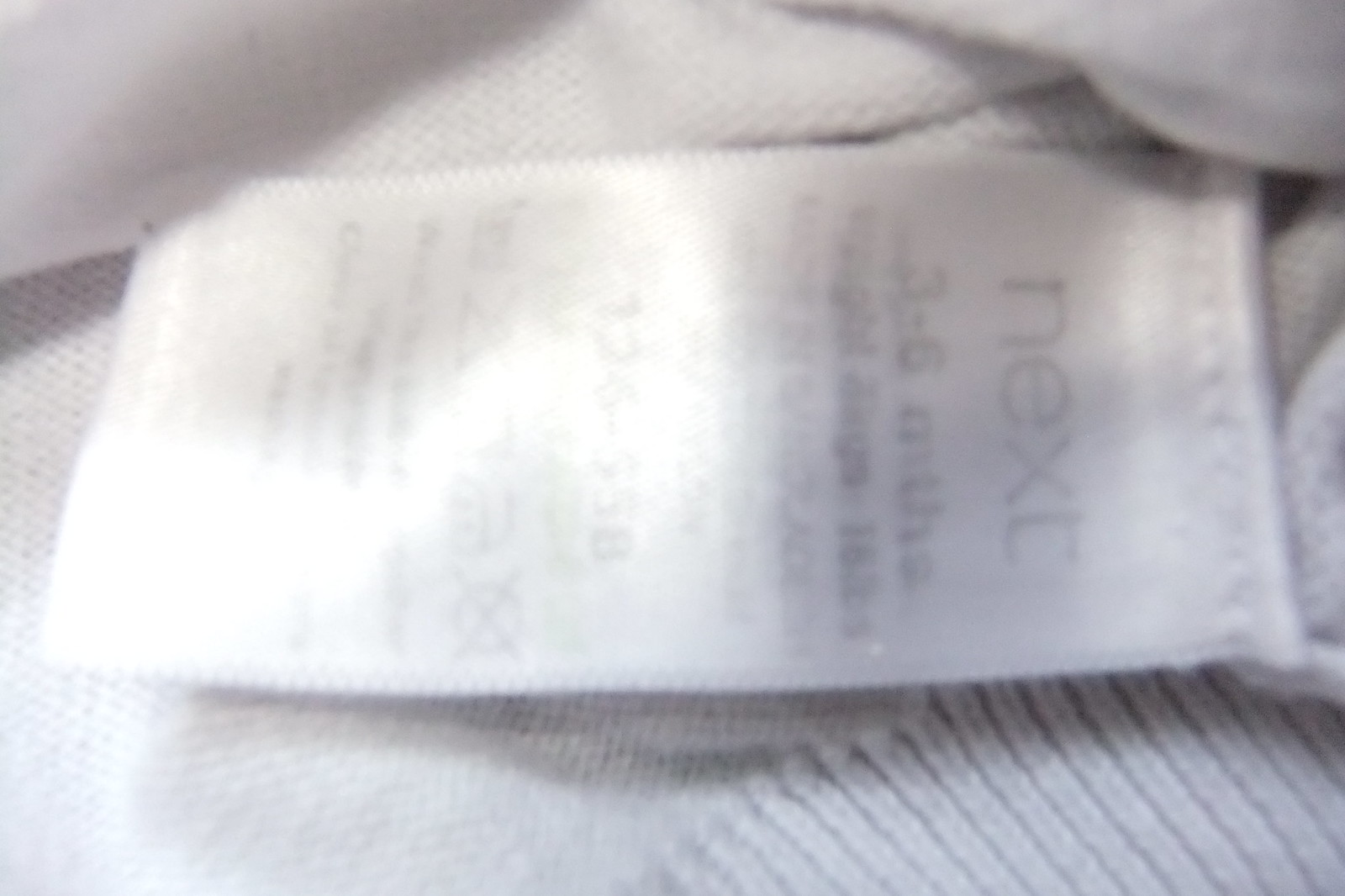In this blurry, close-up photograph, we see a soft, pale white or cream-colored knit sweater for a baby, with a satin tag stitched onto it with white thread. The tag, which appears to be heavily worn and faded from frequent washing, is positioned with the top towards the right and the bottom towards the left. In faded gray letters, it displays the brand name "Next" in capital letters, followed by "3-6 MTHS" and "16 pounds." The majority of the text is nearly illegible due to a bright shadow and significant wear, but some details such as washing instructions can be partially discerned, like no ironing and probably no machine washing, suggesting hand wash. The entire image is dominated by white, with the black printing on the tag being the only other color present.